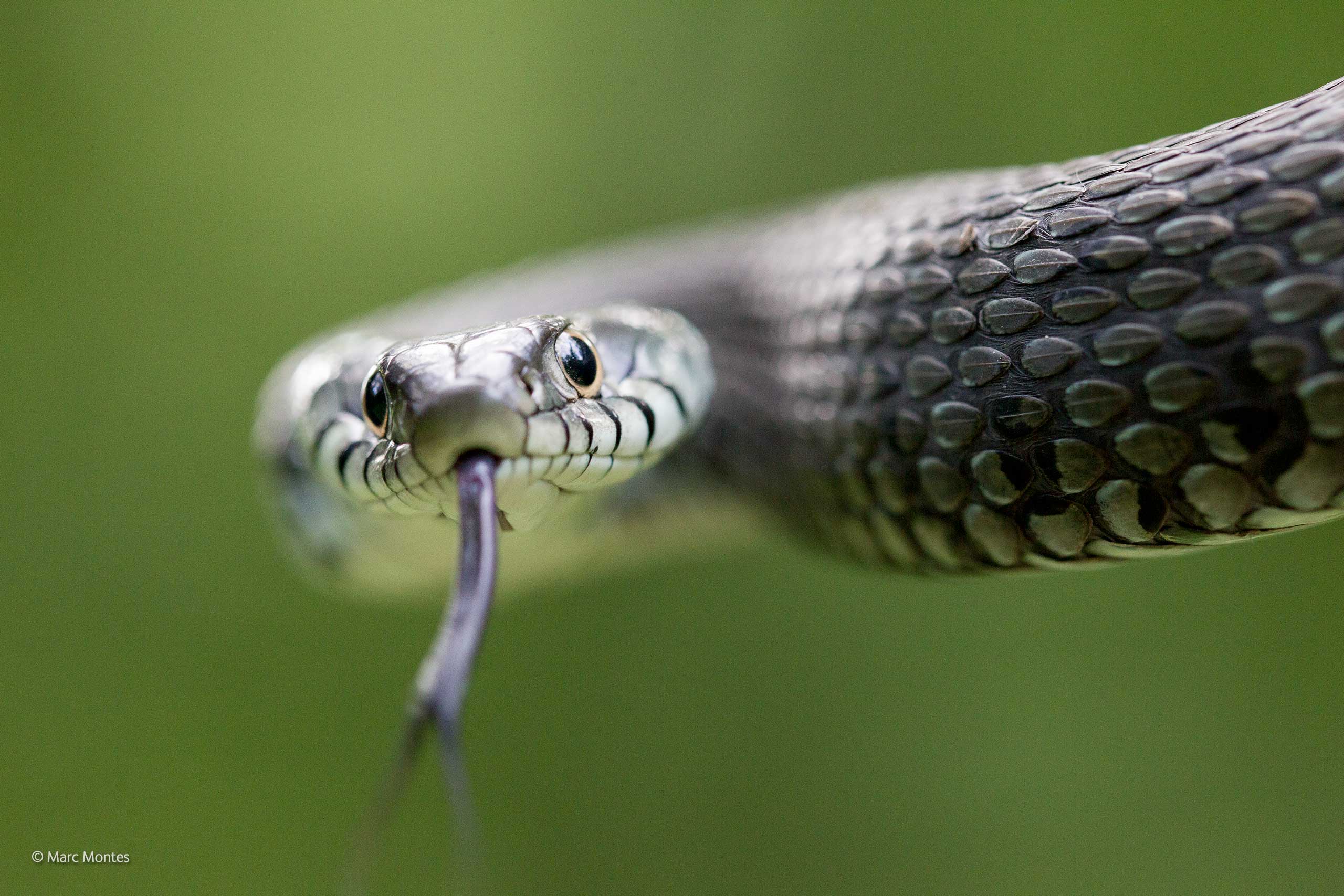This close-up photograph by Marc Montes captures a snake staring directly at the camera with its forked black tongue extended toward the viewer. The snake's textured scales are intricately detailed, winding along its dark grey to black body. Its large, diamond-shaped head appears lighter, with a greenish or cream hue, and features piercing black eyes surrounded by a golden or hazel outline, giving the impression it's about to attack the camera. The background is a uniformly blurred green, adding to the focus on the snake's head, positioned centrally in the frame. A copyright notice for Marc Montes is visible in the lower left corner.